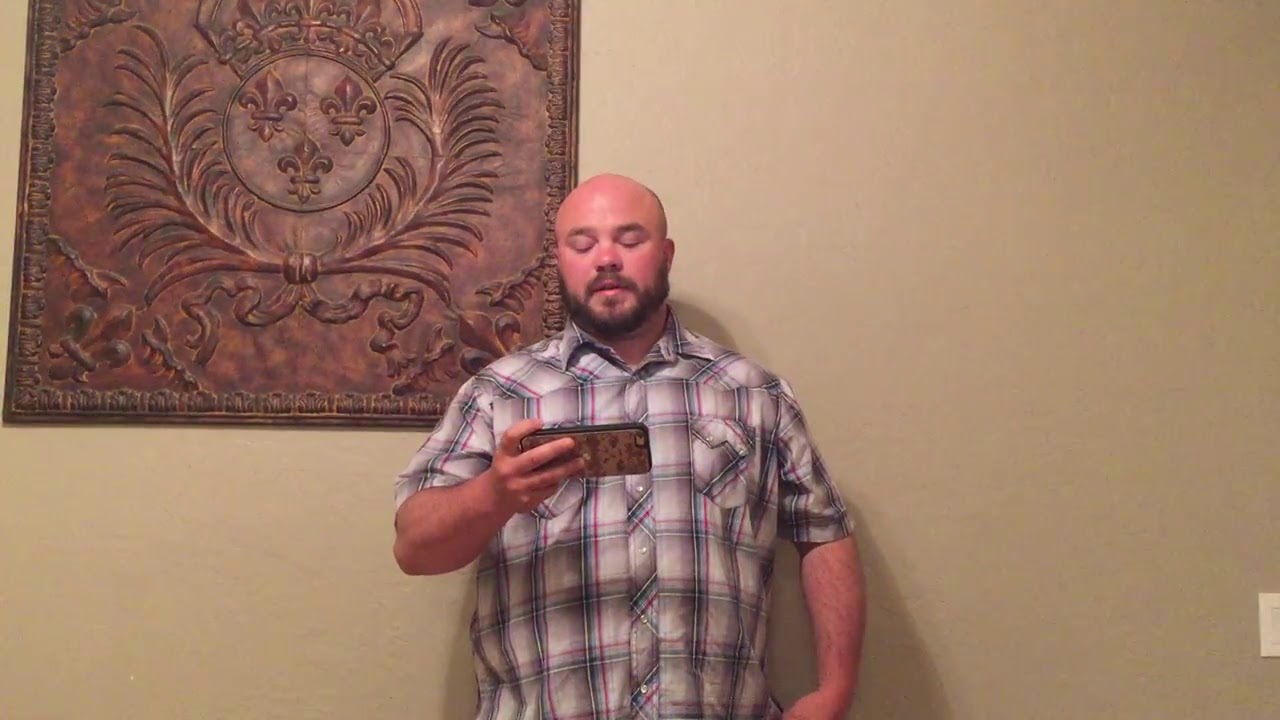In this indoor, landscape-oriented color photograph, a slightly heavier set Caucasian man around 40 years old with a bald head and light brown beard and mustache stands against a light tan wall with a switch cover visible at the bottom. The man, wearing a short-sleeved button-up flannel shirt with a checkered pattern in shades of white, gray, blue, and pink, is the focal point. He holds a cell phone with a sand camouflage-style cover in his right hand and is intently looking down at it. To his right and partially above him on the wall is a large, detailed square metal plaque in hues of bronze and copper. This plaque, featuring a photorealistic representational style, includes an embossed design with a central circle containing three fleur-de-lis and a crown atop. Flanking the circle, two curved feather-like elements extend outward, tied together at the center with a ribbon that hangs down.